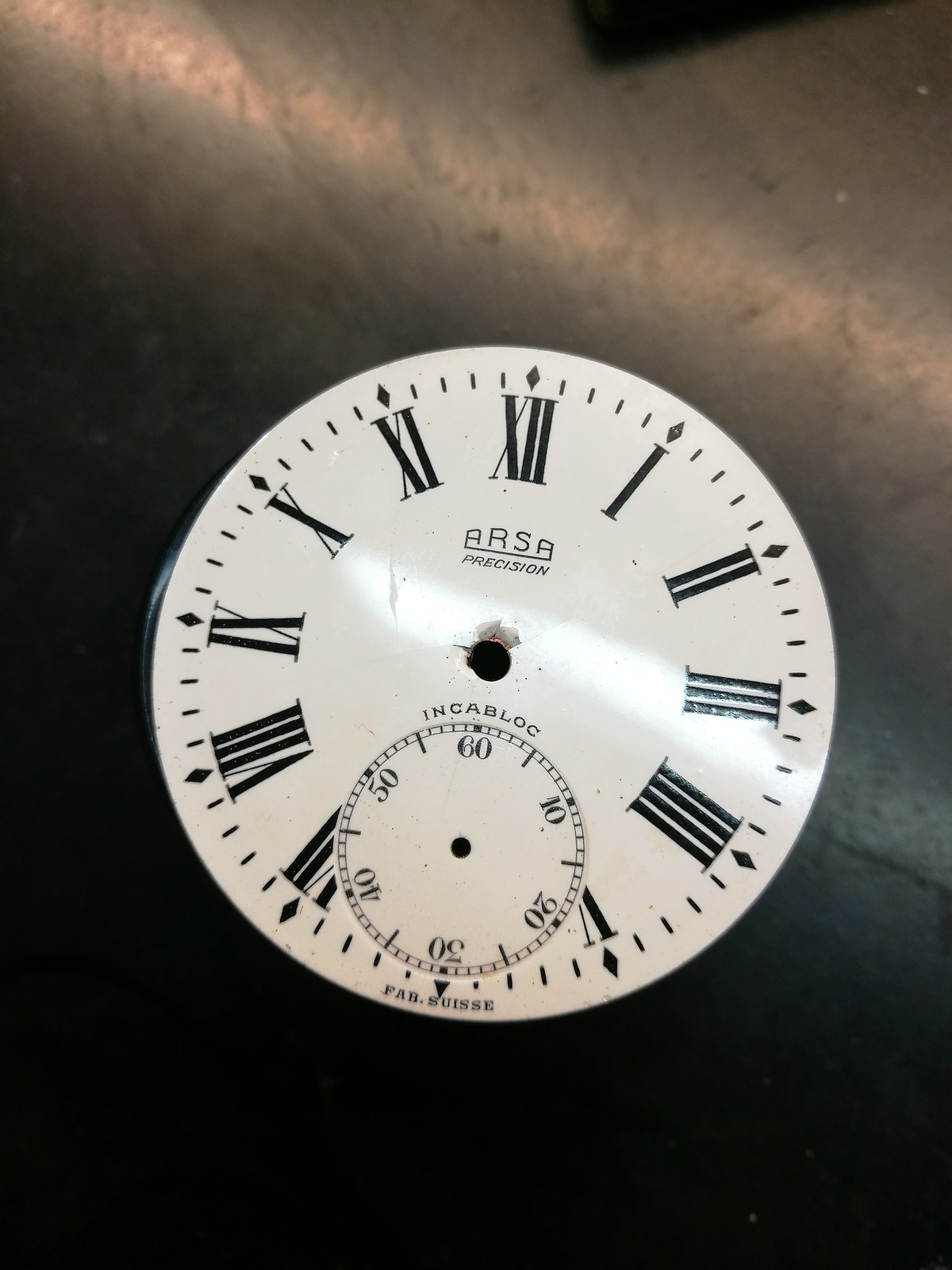The vertically rectangular image features an indistinct background with its lower portion shrouded in black, transitioning to a tan upper section. A subtly dim beam of light traverses from the upper left to the upper center-right of the frame, casting gentle illumination. Dominating the scene is a large clock with a white face, set at a slight tilt so that the number 12 is slanted to the right. The clock's Roman numerals, all rendered in black, are arranged around the face. notable for the absence of clock hands. Positioned at the bottom, where the Roman numeral VI typically resides, is a smaller black circle likely intended for counting seconds. This sub-dial lacks a hand but features a central black spot, with the numbers 60, 10, 20, 30, 40, and 50 marked around its circumference.